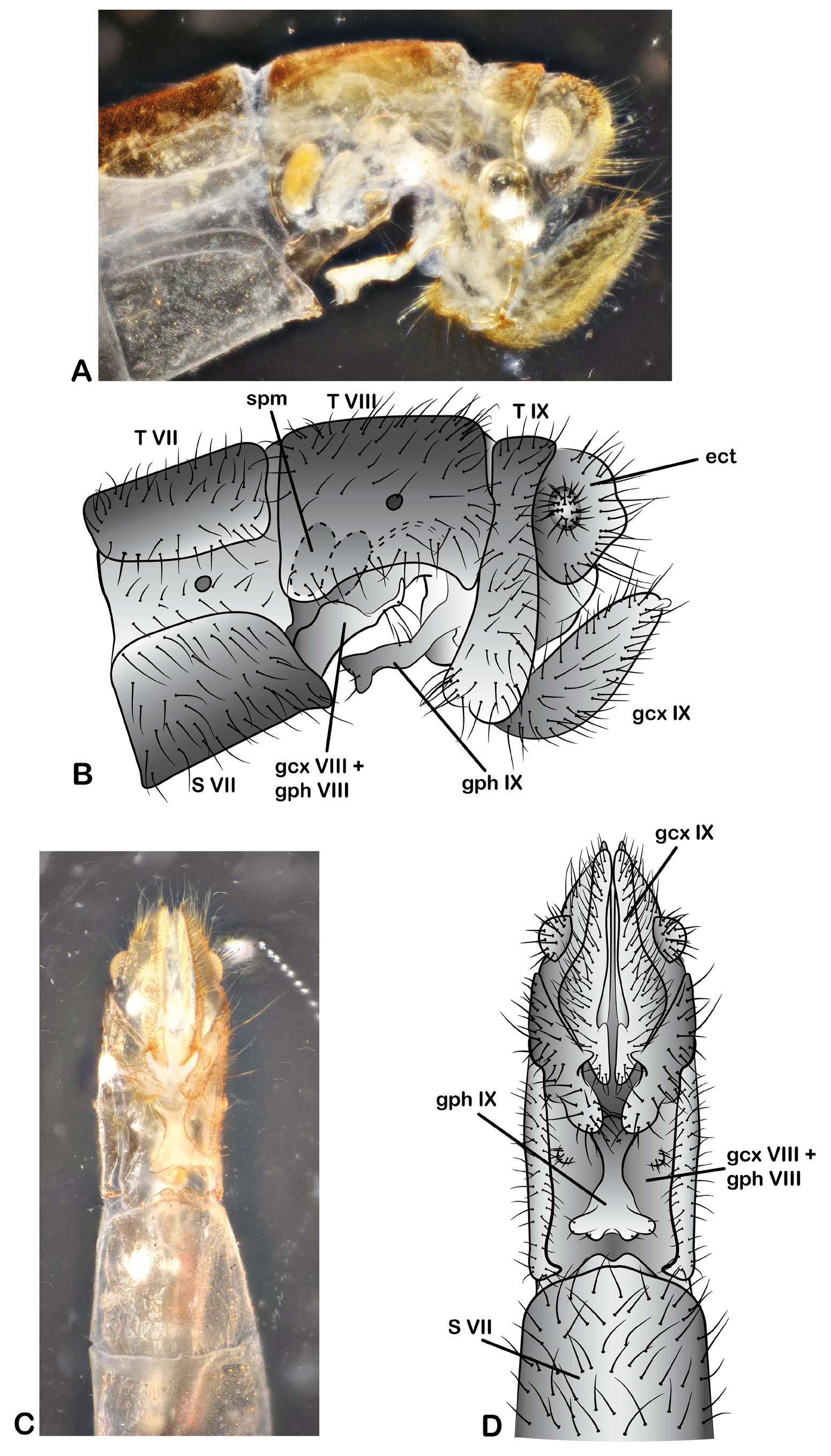The infographic depicts a detailed examination of an unidentified bug or sea creature, possibly captured under a microscope. The graphic is divided into four sections labeled A, B, C, and D. 

- **Section A** features a full-color photograph of the creature, set against a black background, showing its head and upper body. The creature appears to have a furry texture and is colored in shades of brownish-beige.
- **Section B** presents a black and white line drawing of the same creature, also from the side. This diagram highlights the structure of the creature with labeled parts including "TV2," "SPM," "TV3," and "T9," though the significance of these labels is unclear.
- **Section C** shows another full-color photograph, possibly of the lower half of the creature, again with a black background and the same brownish-beige coloration.
- **Section D** mirrors Section B with another black and white illustration of the creature, this time showing the lower parts labeled with "GPH9," "SV7," and "GCXV3."

Both the photographs and drawings are paired, with each photograph having a corresponding detailed illustration, emphasizing the structure and appearance of the creature from different angles. Despite the precision in the visual data, the Roman numeral labels and other text annotations appear cryptic and provide no clear explanatory information.